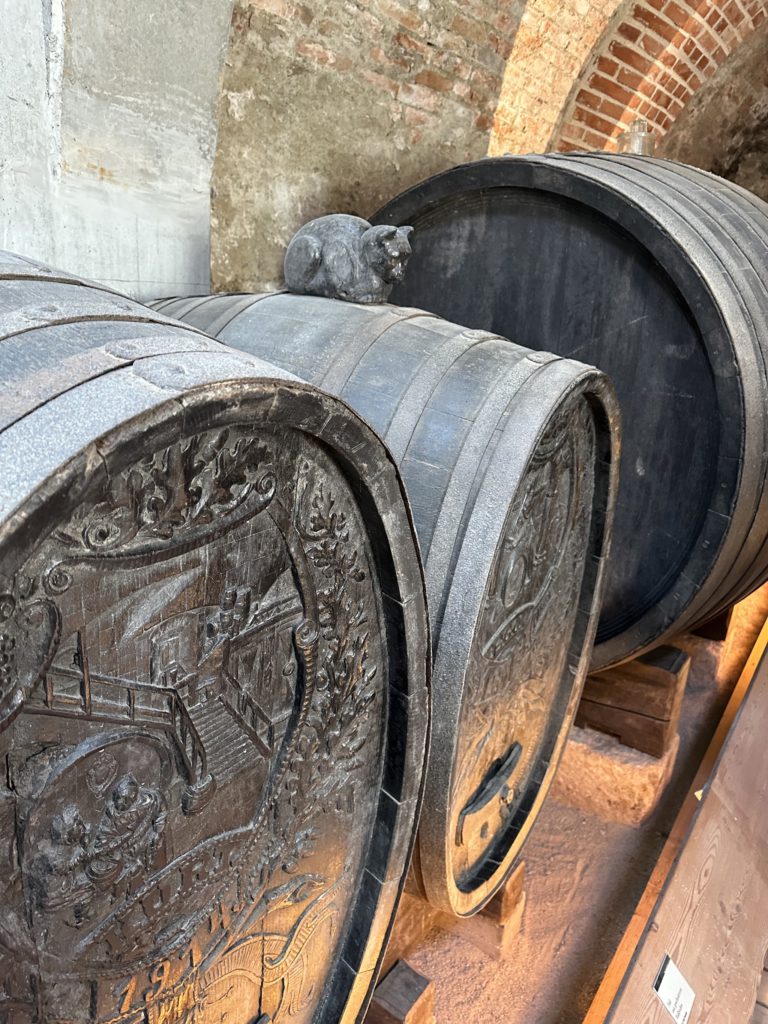The image captures a rustic indoor setting with three large barrels, prominently featured in black and brown hues, accented by belt-like designs. Two barrels lie on their sides, revealing intricately carved lids that depict scenes of winery life, including stairways, people working, and carved trees, along with the number "1914." The third barrel stands upright beside them. Atop the middle barrel sits a wooden cat, adding a whimsical touch to the scene. The background reveals a brick wall transitioning into a concrete surface, under an arch ceiling, bathed in sunlight that highlights certain areas, further enhancing the vintage atmosphere.